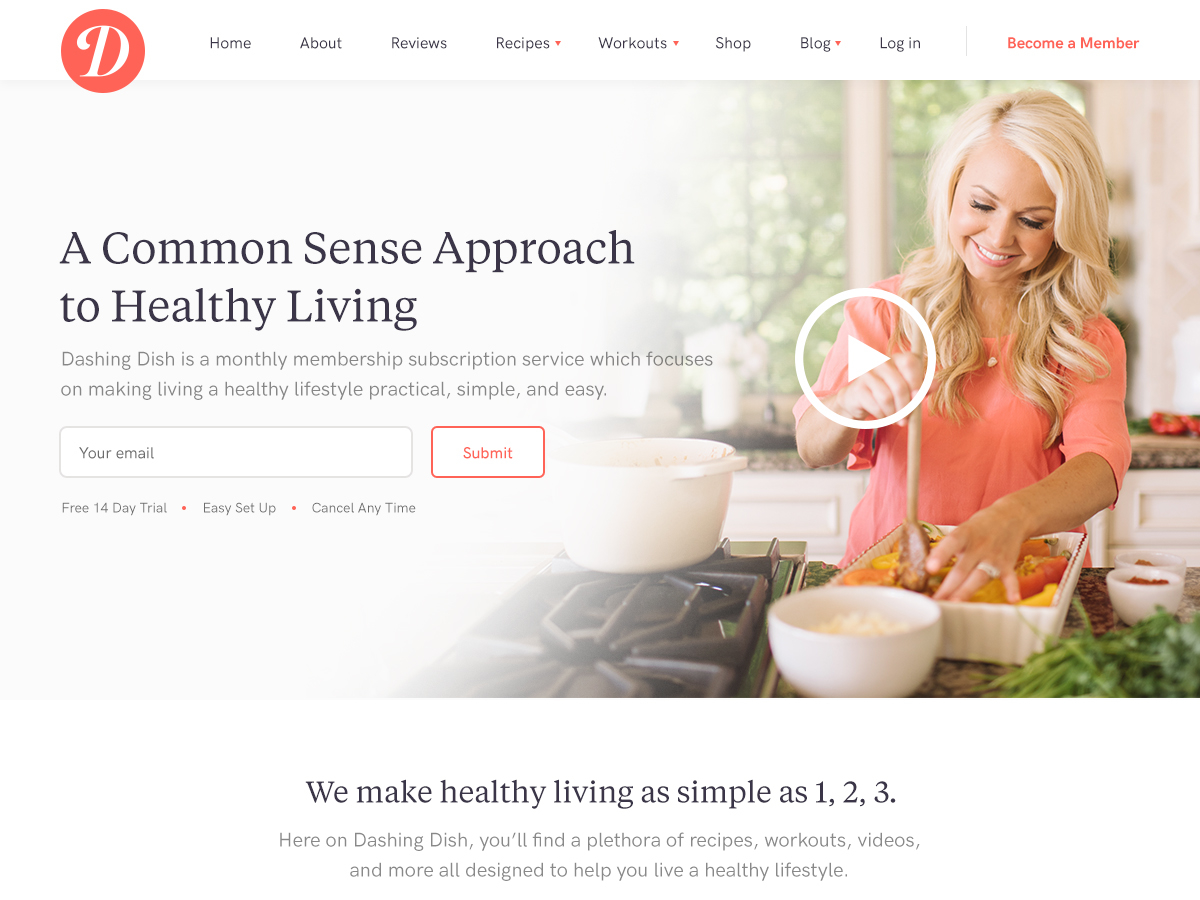The image depicts a vibrant and well-organized cooking website. At the top left corner, there's an orange circle with a white letter "D" inside it. To the right of this icon, a horizontal menu bar displays the categories: Home, About, Reviews, Recipes, Workouts, Shop, Blog, and Login. The words "Become a Member" are positioned at the top right corner in red text. Tiny red heart icons appear next to the categories Recipes, Workouts, and Blog, indicating their popularity or user favorites.

Taking up the center-right portion of the image is a background photo of a woman cooking. She has blonde hair and is wearing a pink blouse. She is captured in the act of cooking, holding a brown wooden spoon, with her left hand actively engaged in the food preparation. On her left ring finger, she is wearing a piece of jewelry, likely a ring.

On the left side of the image, bold text reads, "A Common Sense Approach to Healthy Living." Below this, a detailed description introduces "Dashing Dish" as a monthly membership subscription service dedicated to making a healthy lifestyle easy, practical, and straightforward.